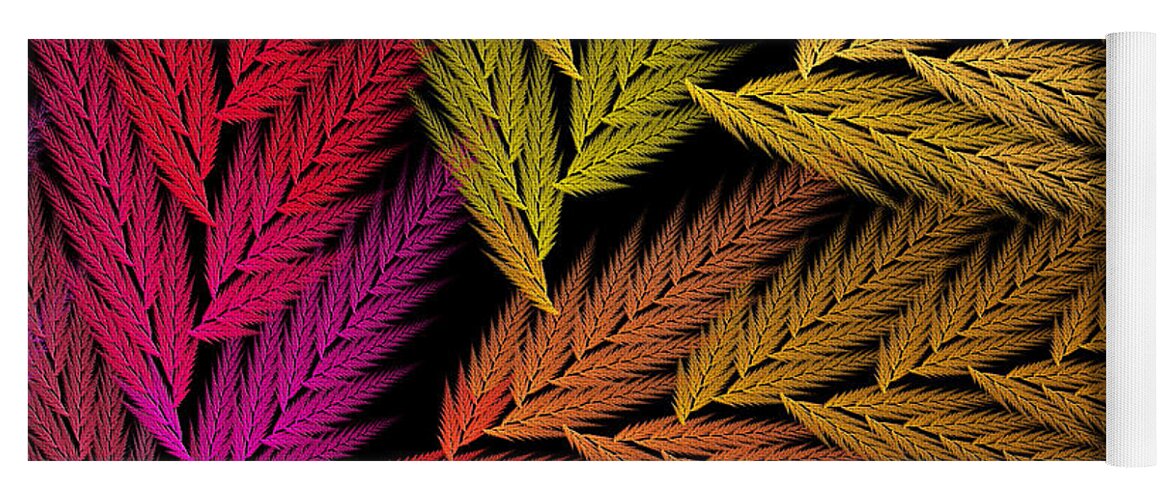The image showcases a rectangular black background adorned with textured, fern-like leaves in a spectrum of vibrant colors that give a stamped appearance. On the left side, you'll find a visually striking array of leaves in shades ranging from lavender and pink to coral, presented in a somewhat fanned-out arrangement. As you move to the right, the leaves transition through a palette of tan, dirty green, and olive green. These leaves are more abundant than their red and pink counterparts on the left. Scattered yet aesthetically pleasing, about 15 branches span the canvas, blending bright hues of pink, orange, and yellow. Highlights include a reddish-pink cluster on the left, lime green leaves at the top center, brown leaves towards the middle, and golden wheat-colored leaves at the bottom right. This vivid and detailed piece would make a captivating wall decor.